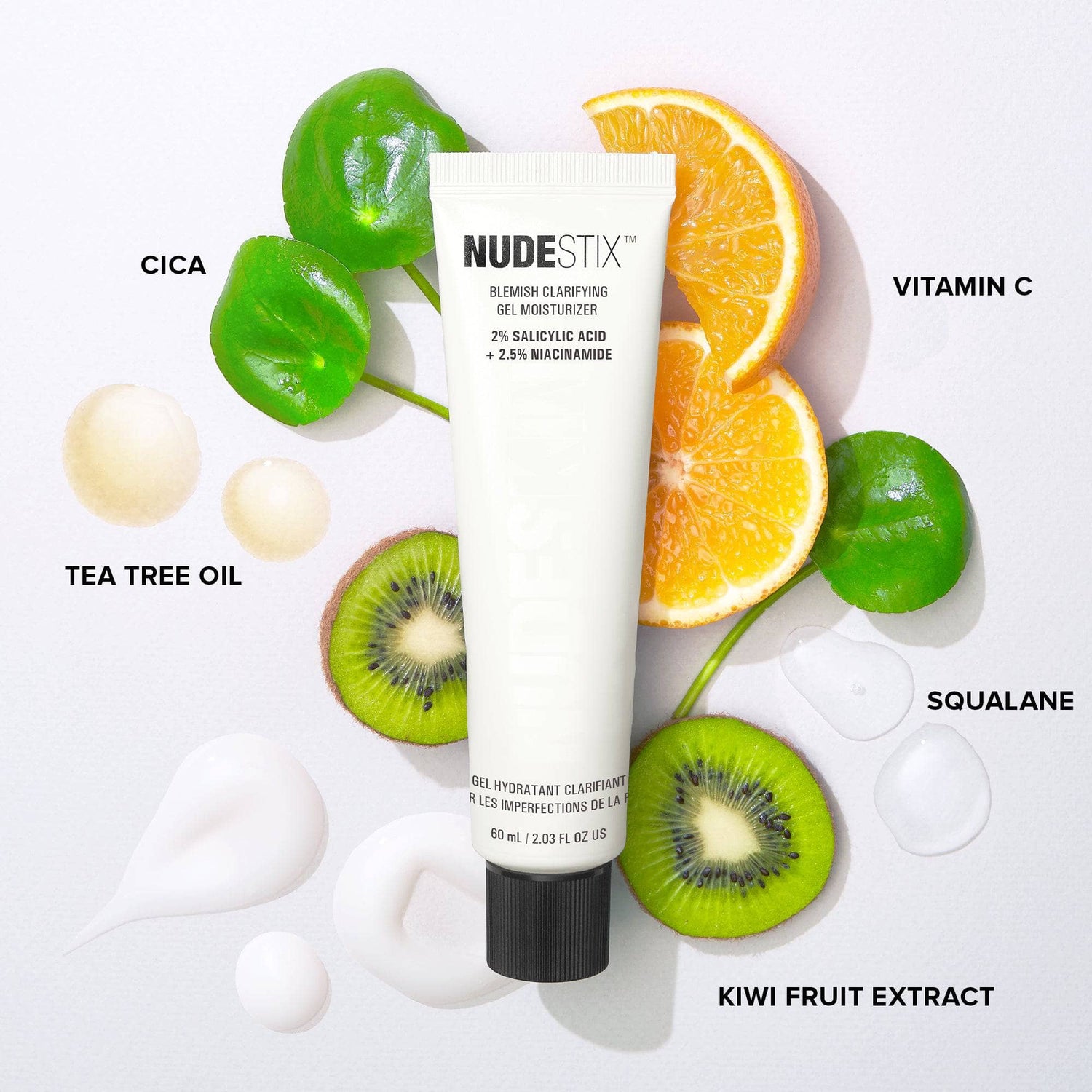This advertisement image features a clear, white background and prominently displays a white tube with black lettering and a black cap. The product, Nude Stix Blemish Clarifying Gel Moisturizer, is emphasized with its key ingredients and benefits labeled. The moisturizer contains 2% salicylic acid and 2.5% niacinamide, designed for blemish control, and is presented in a 60 milliliter (2.03 fluid ounces) tube. Surrounding the product are visual elements representing the core ingredients: glossy green cica leaves, orange slices labeled with vitamin C, droplets of squalane, a slice of kiwi labeled kiwi fruit extract, and amber-colored tea tree oil drops. Additionally, beneath the tube, there is a sample of the moisturizer, showcasing its creamy white texture. These elements combined illustrate the natural and beneficial components of the product, creating a clean and appealing overall aesthetic.